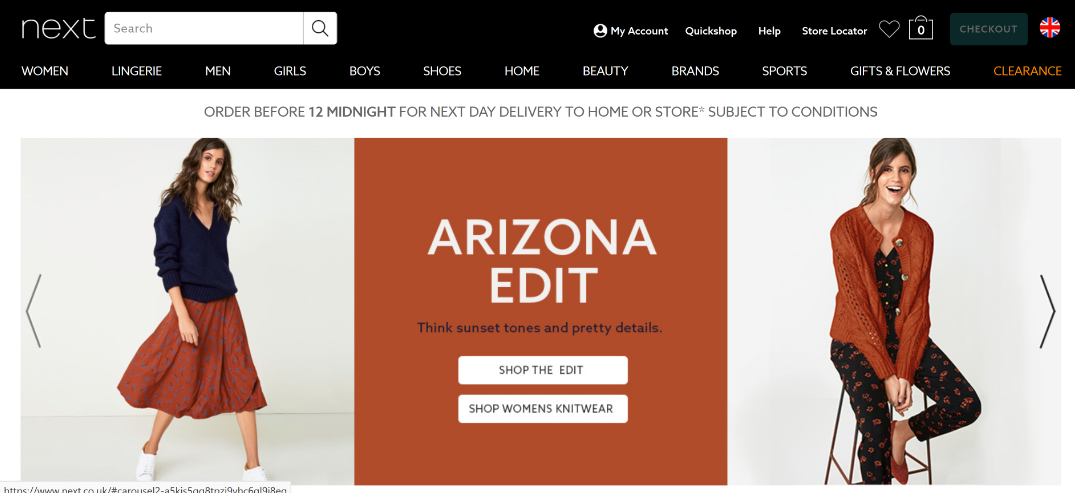A detailed screenshot of a clothing retailer's desktop website interface displayed in a browser. The top of the page features a sleek black banner with the word "Next" prominently displayed. Directly following are a search box and an icon resembling a microscope. The navigation bar includes options reading: "My Account," "Quick Shop," "Help," "Store Locator," an icon of a heart, "Shopping Bag," "Checkout," and a British flag situated on the far right.

Beneath this banner, a secondary horizontal menu presents various categories: "Women," "Lingerie," "Men," "Girls," "Boys," "Shoes," "Home," "Beauty," "Brands," "Sports," "Gifts & Flowers," with "Clearance" highlighted in orange on the right.

Below the menus, a gray banner reads: "Order before 12 midnight for next day delivery to home or store, subject to conditions."

On the left side of the image, a Caucasian girl with long, flowing black hair is depicted walking. She wears a navy blue V-neck sweater with sleeves slightly pushed up and a red burgundy skirt that puffs out slightly and falls to her knees. She completes her casual outfit with white tennis shoes.

In the center of the image, "Arizona Edit" is written in white font against an orange background.

To the right, a woman is seated on a stool, contributing to the overall aesthetic of the website's design.